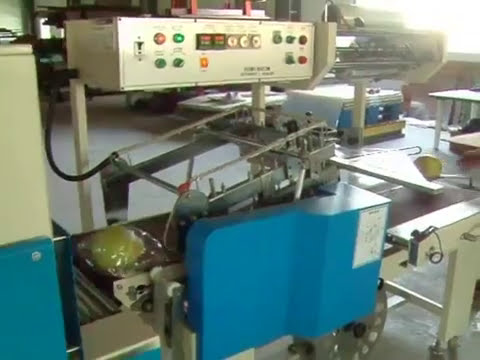The image captures a detailed scene inside a control room filled with various machinery and electrical equipment. Central to the image is a large machine featuring a prominent white control panel that includes a series of red and green dials and buttons of various sizes. Positioned on top left are a red button and a green button, followed by two green unlit buttons underneath, and a row of two black switches and three white knobs to their right. Next to these, there are three additional knobs—two green and one red—mounted on a steel support structure, with a small conveyor belt underneath, guarded by a blue barrier. 

To the left side of the image, there is a dresser or drawer with a cream or beige top and a matching light blue bottom, echoing the blue panel towards the center of the image. Additionally, gray and white components are noticeable, connected to either an output or input panel, with a partial blue covering. In the background, other pieces of equipment and a table can be seen on the right side. A soft yellow or white light, possibly from a window, streams in from the top right corner, illuminating the intricate setup of the control room.